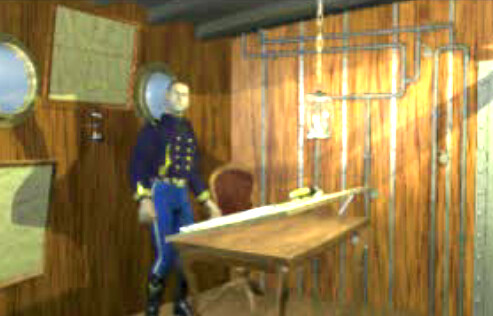In this slightly blurry image, a man in a military uniform stands inside a room, suggesting a maritime setting. He is positioned next to a small wooden table, alongside a high-back chair featuring a wooden frame and dark brown cushioned seat. The backdrop consists of wood-paneled walls with a navigational map prominently displayed on one of the panels. Flanking the map are portholes through which a bright blue sky is visible, reinforcing the impression that the setting is aboard a ship.

The man is dressed in a distinctive short navy blue jacket adorned with double rows of gold buttons on the front and gold detailing at the cuffs. His lower attire includes royal blue tights with white stripes running down the sides, paired with boots completing his military ensemble. To his left, there is a larger window draped with sheer orange and gold curtains through which sunlight streams, enhancing the room’s ambiance. On the small table in front of him lies a rolled-up piece of paper, adding to the scene's historic and nautical character.